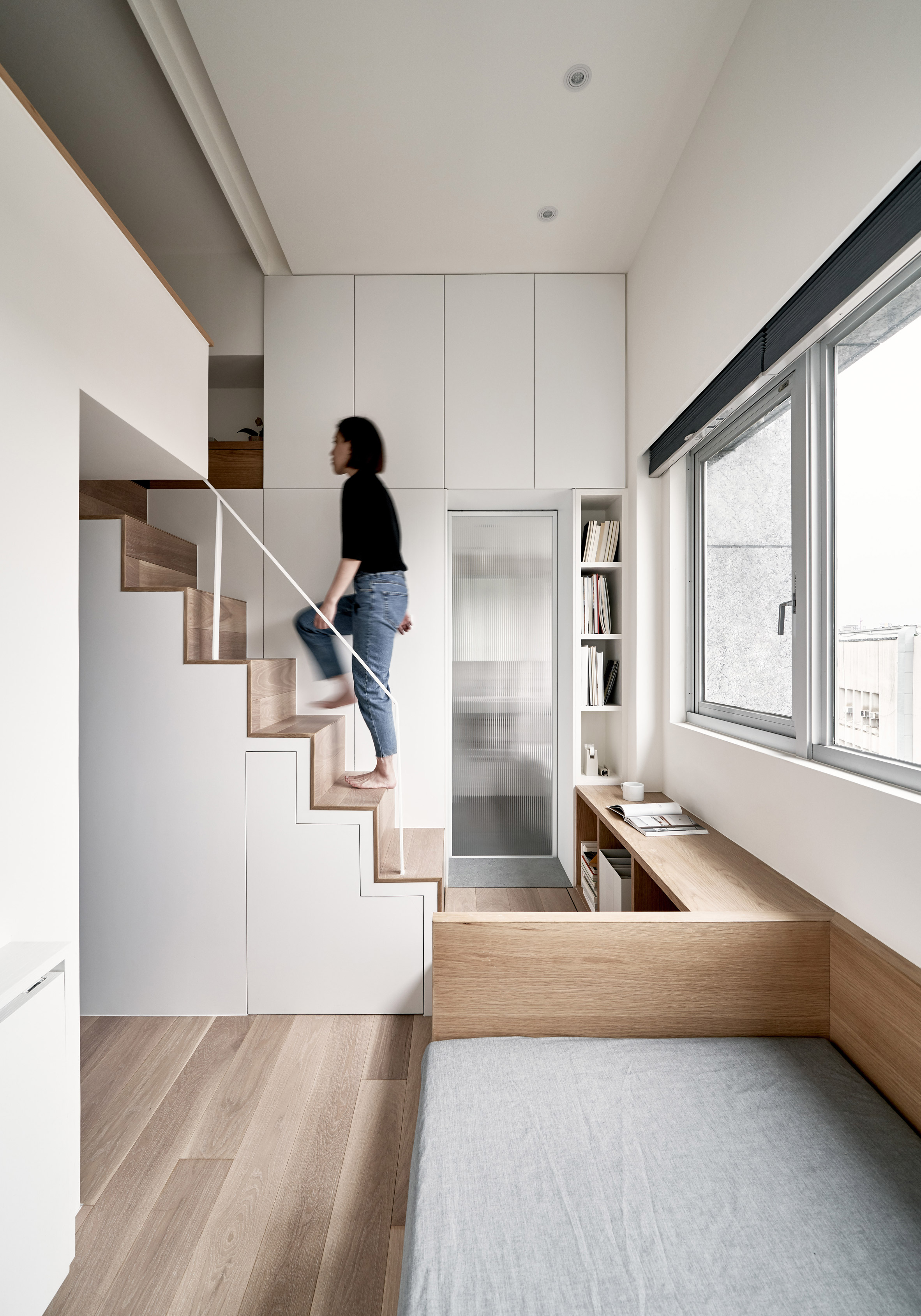This image shows a compact, minimalist living space that could be a small apartment or a tiny home, characterized by its white walls and tan wood accents. On the left side, there are large, undressed windows with possible shades above them, featuring a crank handle on one window. Underneath these windows runs a tan wood shelving unit, partially hidden by a white or tan basket that adds to the clever storage solutions.

Dominating the back wall are four white closet panels that extend about a third of the way down the wall. Below these closets, a sliding glass door reveals a small office nook or bookcase behind it. 

In the foreground, on the right, a cozy bench seat with a light wood frame and a gray cushion faces the viewer. Adjacent to the bench, a step-up area with matching laminate wood flooring extends toward a set of steep stairs. 

At the center of the composition, a woman, barefoot and dressed in a black short sleeve top and blue jeans, ascends these steep stairs. She has dark, shoulder-length curly hair and some facial hair. The stairs likely lead up to a loft or second-floor area. The architectural design of this space, combined with its clean, uncluttered aesthetic and warm wood tones, creates a cozy and efficient living area.